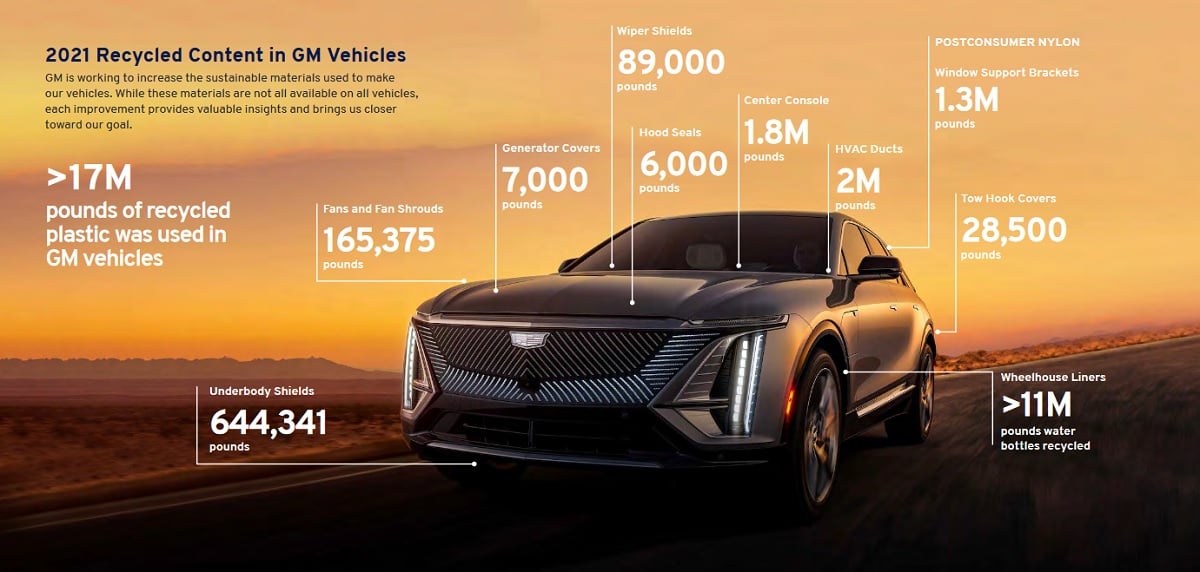In this captivating car advertisement set against an evocative sunset with rich orange-yellow and pinkish hues, a dark gray vehicle with black accents stands prominently on a road, appearing to drive out of a scenic desert landscape. In the top left corner, bold black text reads "2021 Recycled Content in GM Vehicles," followed by a description detailing GM's commitment to increasing sustainable materials in their car manufacturing process. The ad highlights a significant achievement, noting, in white text, that more than 17 million pounds of recycled plastic have been utilized in GM vehicles. Various white callout labels with arrows point to specific parts of the car, such as the generator covers, wiper shields, hood seals, center consoles, HVAC ducts, post-consumer nylon, tow hook covers, wheelhouse liners, underbody shields, and fan and fan shrouds. For instance, the wheelhouse liners alone incorporate over 11 million pounds of recycled water bottles. This detailed representation stresses GM's innovative steps towards sustainability, underlined by striking visuals and data that accentuate the integration of reused materials into the car’s design.